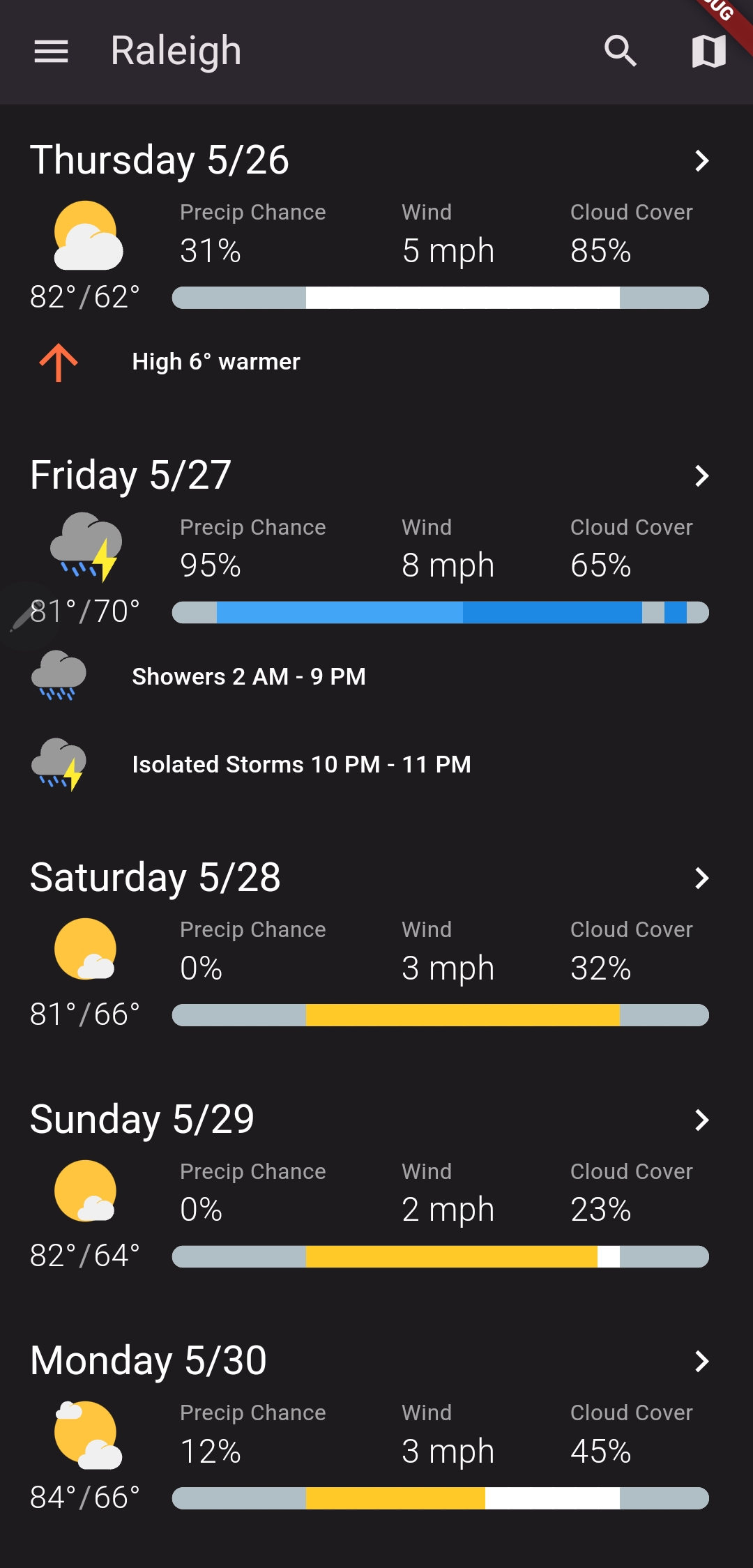This mobile screenshot displays a weather forecasting app interface in detail. At the top left corner is a menu icon, followed by the word "Rally" in white letters. On the far right, there are a magnifying glass for search functionality and a flag icon. Below this top navigation bar, the app presents a vertical list of days, each encapsulated in its own box providing an overview of the weather forecast.

Starting with the day labeled "Friday, 5/27," the box prominently shows a storm cloud icon with a lightning bolt, indicating thunderstorms. Below the icon, the high and low temperatures for the day are displayed. To the left of the temperatures, important weather metrics are listed, including the chance of precipitation, wind speed, and cloud cover percentage. A horizontal blue bar represents the duration of expected rainfall, with specific hours of anticipated rain detailed just below it.

The subsequent day, "Saturday, 5/28," follows the same structured format, providing consistency across the forecast for multiple days. Each day's forecast summary features a small white arrow on the right side of the box, inviting users to expand for a more detailed view of the weather conditions.